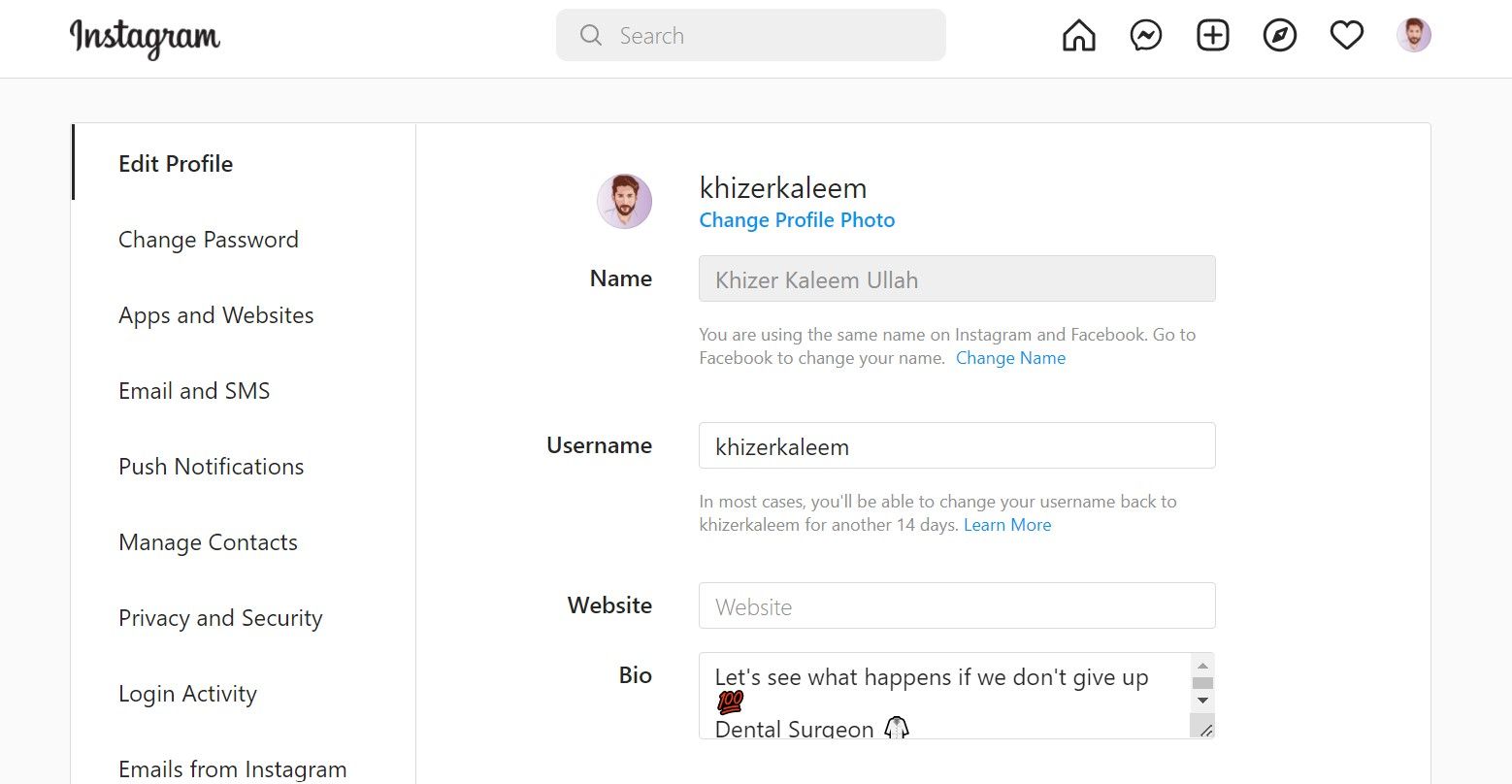**Instagram Profile Overview Screenshot**: 

This image captures a detailed view of an Instagram profile settings page. At the top left, the iconic Instagram logo is visible. Adjacent to it, there is a search bar, followed by a row of icons - a home icon, a messaging icon, a "plus in a box" to add content, a compass icon for exploration, a heart icon for notifications, and finally, a profile picture of a light-complexioned individual with dark hair and a beard, encapsulated in a circle.

Below the logo, a list of options is displayed: 
- Edit Profile 
- Change Password 
- Apps and Websites 
- Email and SMS 
- Push Notifications 
- Manage Contacts 
- Privacy and Security 
- Login Activity 
- Emails from Instagram 

In the central part of the image, the profile owner’s name, spelled as "K-H-I-Z-E-R-K-A-L-E-E-M" in bold, is prominently displayed alongside another circular profile picture. Below, there is an option in blue to "Change Profile Photo."

The name field shows "K-H-I-Z-E-R  K-A-L-E-E-M  U-L-L-A-H" in a gray data field, followed by a notification stating, "You are using the same name on Instagram and Facebook. Go to Facebook to change your name," with a blue prompt to "Change Name."

Lastly, the username "K-H-I-Z-E-R-K-A-L-E-E-M" is shown in a white data field, accompanied by a message indicating that in most cases, the username can be reverted within 14 days, with an option to "Learn more."